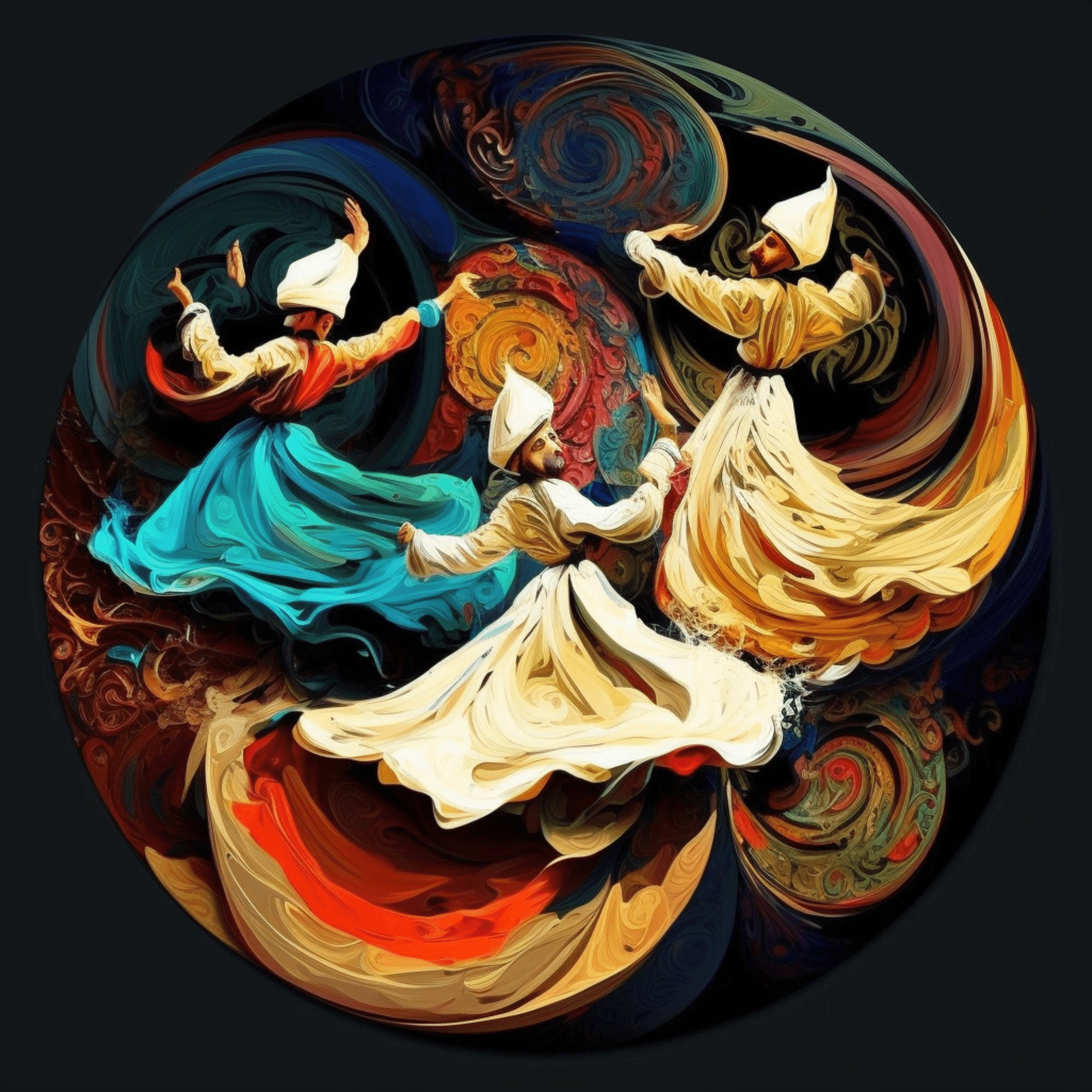The image is a detailed painting with a predominantly black background. At the center, there are three men in cultural costumes, likely whirling dervishes, each wearing white turban-like hats. These figures are depicted in dynamic poses as if dancing, contributing to the circular motion evident in the image. The man at the upper left wears a beautiful turquoise robe and raises his hands in the air. In the middle, a figure in a white flowing gown and a beard looks back. On the upper right, another dancer in a cream-colored gown extends his arms outwards. Their flowing robes blend seamlessly into a swirling design of red, green, blue, and orange hues, which forms a large, encompassing circle. This artistic rendition, rich in vibrant colors and circular motifs, captures both the dance and the intricate, spiraling patterns, creating a mesmerizing and immersive visual experience.